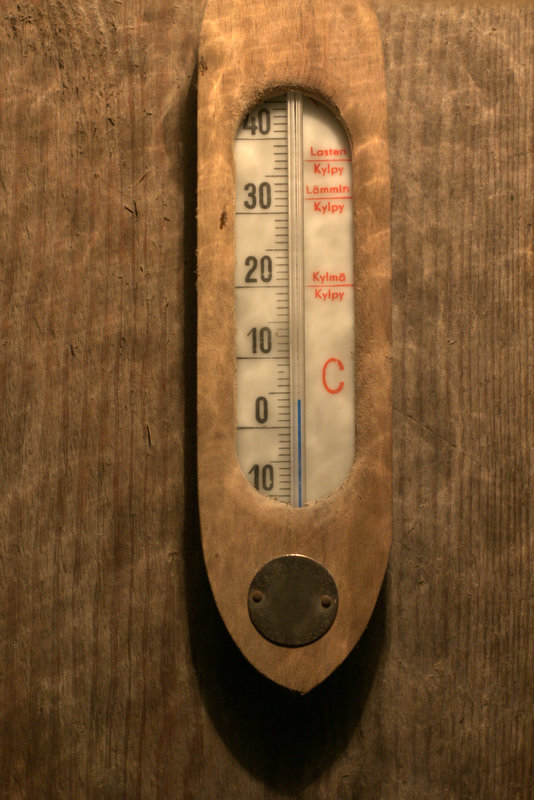This photograph features a vintage thermometer encased in a wooden frame. The craftsmanship of the wood highlights the antiquity of the piece. The thermometer measures temperature in Celsius and includes inscriptions in a language that appears to be either Swedish or Finnish, indicating its likely Scandinavian origin. This unique, historical instrument reflects the intricate design and functionality of past eras.